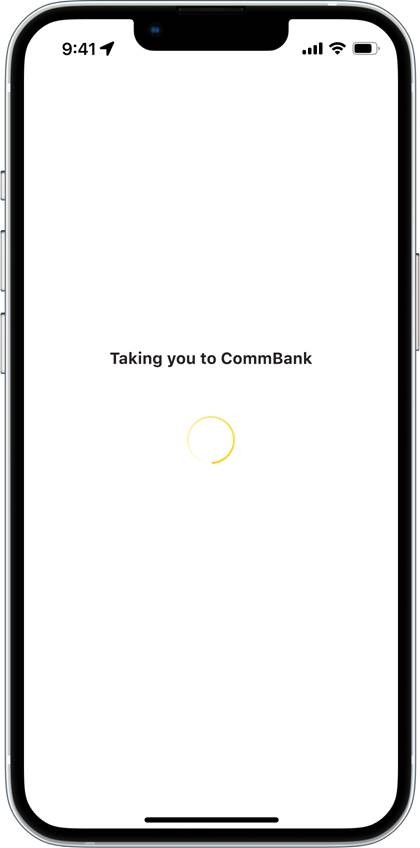The image depicts a cell phone with a metallic finish, likely silver or white. On the upper left corner of the screen, the time "9:41" is displayed in black text, while the upper right corner shows signal bars for cellular, Wi-Fi, and a mostly charged battery icon. The phone's screen has a white background.

In the center, there is a message in black font that reads, "Taking you to Com Bank," with the letters "C," "O," "M," and "B" particularly emphasized in uppercase. Below this message, a yellow loading circle is visible. The circle appears to be in motion, captured in a particular frame where parts of it are light yellow, almost white, and other segments are a darker yellow.

At the bottom of the screen, there is a prominent black line, accompanied by a thinner black border framing the entire display. The surrounding area beyond the phone is a consistent white background, blending seamlessly with the phone's screen, giving the appearance of an almost borderless design. The overall color scheme of the image is composed primarily of black, white, and yellow, with no gray tones present. The display indicates that the phone is in the process of loading the "Com Bank" app or website, with no additional navigation elements visible.